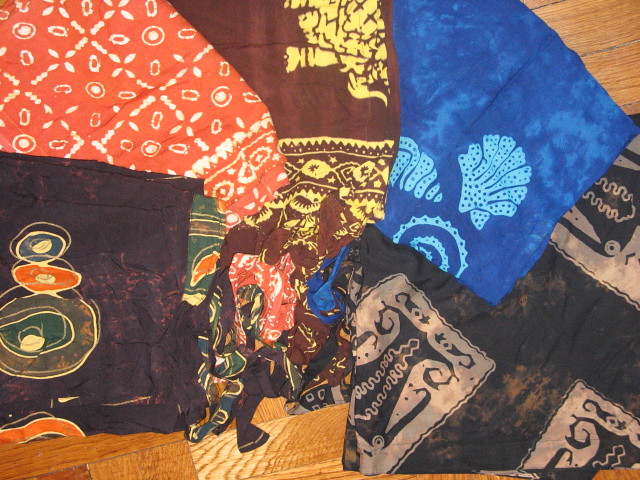This detailed color photograph depicts an array of assorted fabrics strewn across a wooden floor. The image, slightly wider than it is tall, features six distinct fabric patterns, each with unique designs and color schemes, arranged in an overlapping, haphazard manner. 

At the top left, there is a red scarf with an intricate white pattern. To its right, a brown piece adorned with a yellow decorative motif captures attention. Below this, a blue fabric showcases light blue seashells in a batik style. On the bottom left, another brown piece features a geometric design. Centrally nestled, a crumpled scarf appears to feature a more abstract or floral pattern, adding to the visual complexity. Lastly, at the bottom right, a black fabric displays white geometric patterns within squares.

The wooden floor, visible at the upper right and bottom left corners, comprises light to medium tan planks with darker brown variations, suggesting a natural, oak-like texture. The photograph is well-lit, favoring natural light, which brings out the vividness and detail of each fabric's design. The overall composition, highlighted by the varied patterns including seashells, geometrics, and abstract motifs, evokes a sense of artistic randomness and tactile richness.